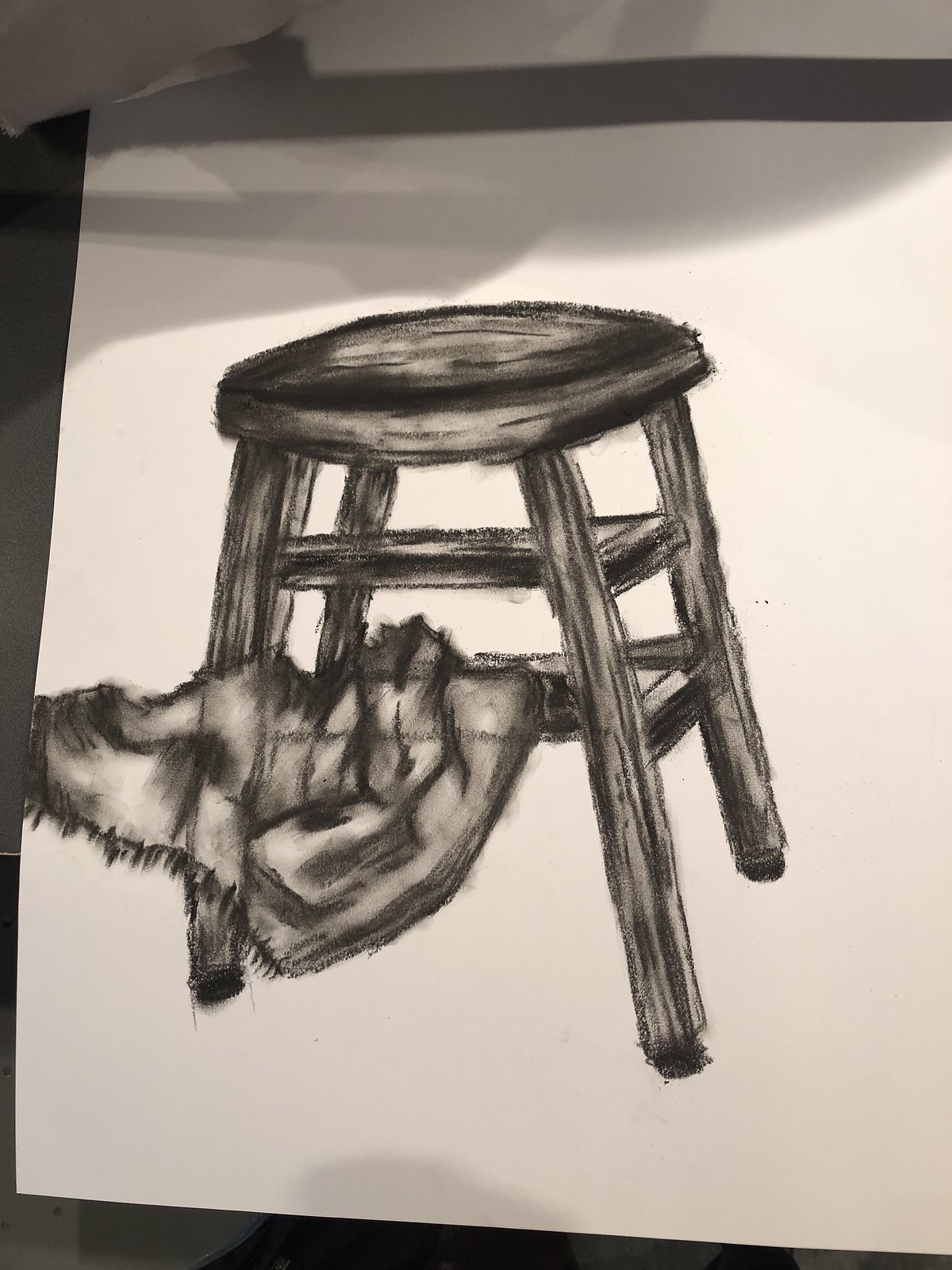This is a detailed charcoal or thick pencil drawing on a tilted white sheet of paper, depicting a wooden bar stool with a round seat. The seat displays circular grain patterns suggesting it is made from wood, and the stool's edges and support beams are shaded darker. The stool is supported by four elongated legs, three of which are visible, with black tips at the bottom. Halfway down the legs are horizontal rungs, accompanied by additional rungs just beneath the seat. Draped over the top of the stool is a fabric item, characterized by its wrinkled texture and fringed bottom, flowing towards the left side of the image. The presence of a shadow at the top hints at the photographer leaning over the light source. The entire scene rests on a gray table.